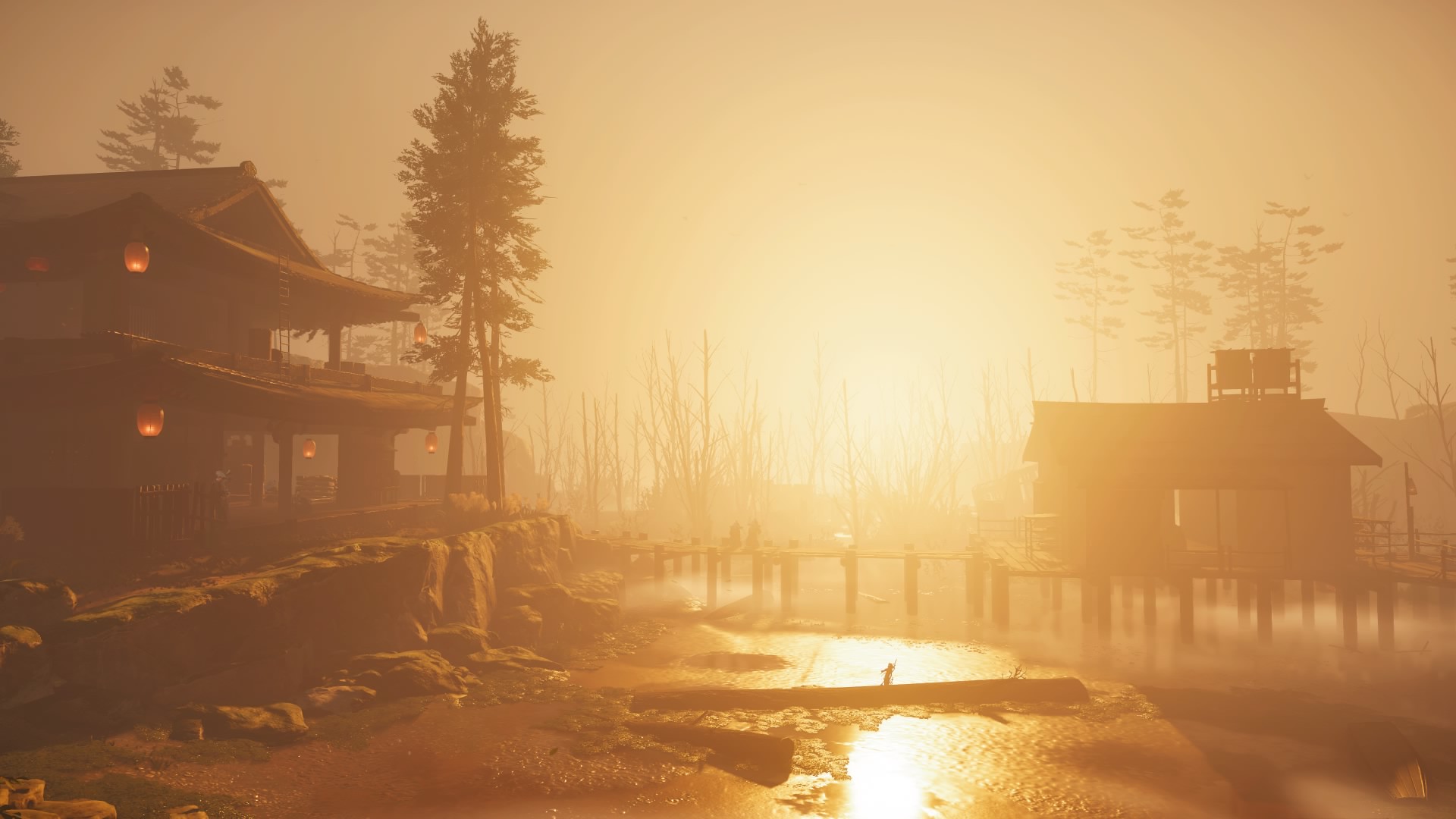This artistic landscape image, likely computer-rendered, depicts a serene morning scene with a yellowish, sunlit mist gradually lifting. A shallow, undulating creek flows through the center of the composition, reflecting the soft morning light. On the left, an Asian-style pagoda with two levels and a triangular rooftop stands perched on a rocky edge. This pagoda is adorned with traditional paper lanterns. To the right, another cabin, elevated above the creek on stilts, is connected to the pagoda by a wooden pier. Tall, spindly pine trees surround the structures, adding to the tranquil atmosphere. The overall scene is suffused in hues of orange, dark brown, and light brown, emanating a warm, peaceful vibe typical of dawn.